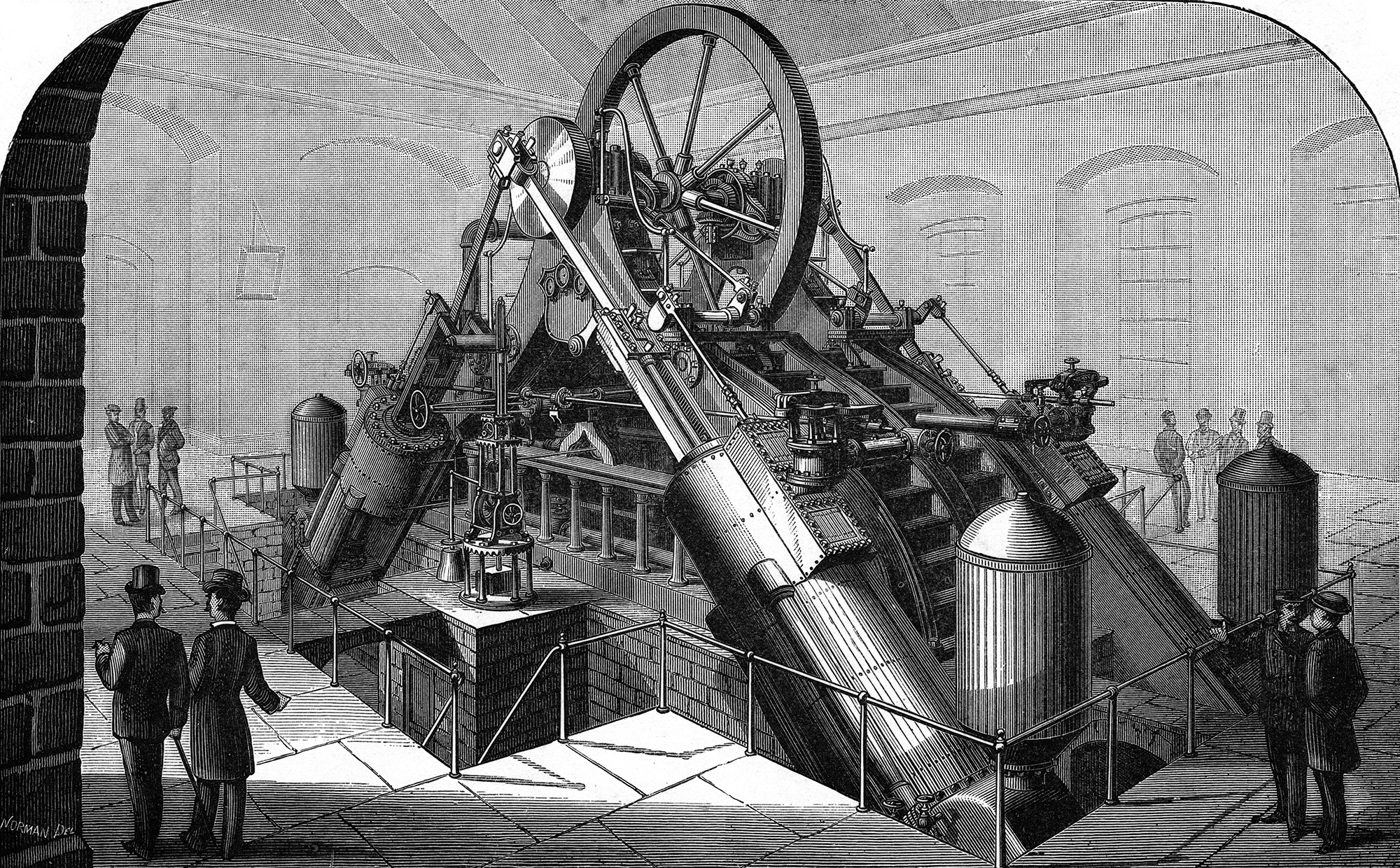This detailed black-and-white drawing by Norman Dell depicts a massive steam machine set within an expansive room with a tall ceiling and multiple archways leading to windows. The focal point is the intricate machine, positioned in a lowered area of the room with stairs leading down to it. The steam machine features prominent dual cylinders positioned at 45-degree angles, connecting to a large flywheel with several spokes at the top center. Below the flywheel, a complex arrangement includes gears and possibly a water wheel. Surrounding the machine are several gentlemen in suits and hats—some are standing and chatting, seemingly admiring the industrial marvel, while others are walking about. The room’s lightly drawn elements, including the silhouettes of the factory's back walls and windows, contrast with the darker, detailed shading of the steam machine, enhancing its prominence in the scene.